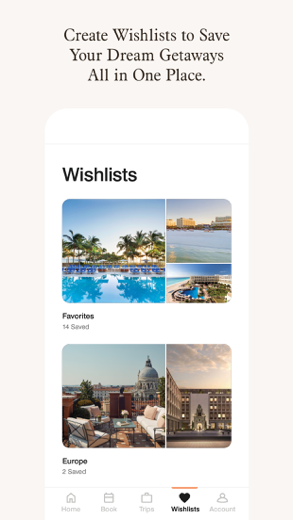In this image, the central focus at the top reads, "Create a wish list to save your dream getaways all in one place." Below this, the image depicts a webpage with a white background, prominently displaying the word "Wish List" in bold black text at the top. 

Underneath "Wish List," there's a section titled "Favorites" with a note indicating "14 saved" items. Accompanying this section, within a bordered box, are thumbnail images of vacation spots. The left image displays a tranquil, blue swimming pool bordered by palm trees. To the right, two images are stacked vertically: the upper image features a serene ocean view with large buildings in the background, while the lower image showcases another pool area encircled by lush trees and rocky formations.

Further down, there's another section labeled “Europe,” noting “2 saved” items. This section also contains a box with images: the left image shows chairs arranged to face a cityscape, and the right image highlights a large, ornate fountain situated in front of an architectural masterpiece.

At the bottom of the webpage, five icons represent various categories: from left to right, they are labeled "Home," "Book," "Trips," "Wish List," and "Account."